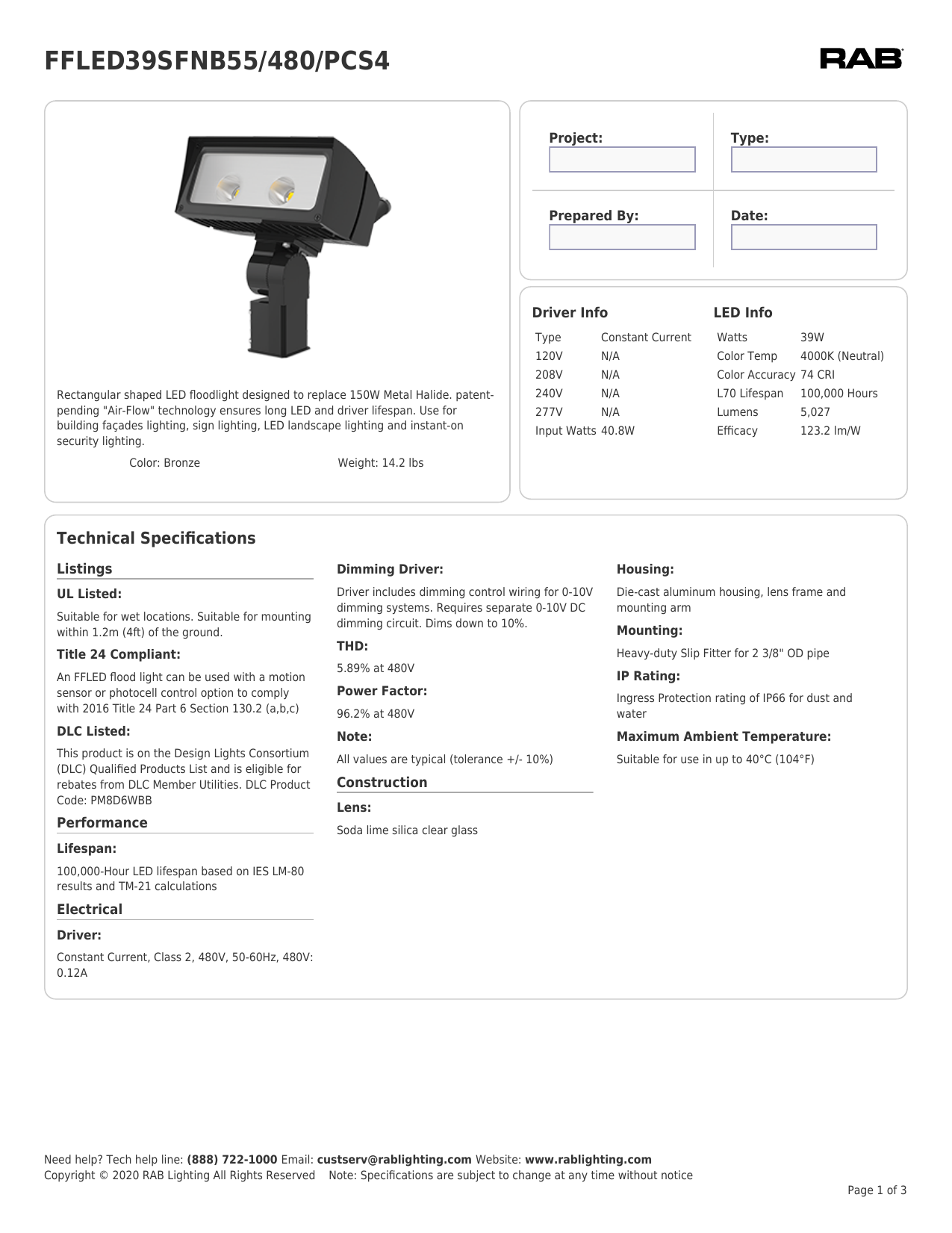**Detailed Product Description for RAB LED Floodlight Model FFLED39SFND55-480-PCS4**

---

**Product Overview:**
- **Model:** FFLED39SFND55-480-PCS4
- **Brand:** RAB

**Visual Description:**
- This image showcases a high-performance, rectangular-shaped LED floodlight designed to replace the traditional 150-watt metal halide fixtures.

**Key Features and Technology:**
1. **Patent-Pending Airflow Technology:** 
   - Ensures a long lifespan for both the LED and the driver.
2. **Design Applications:** 
   - Suitable for building facades lighting, sign lighting, LED landscape lighting, and instant-on security lighting.
3. **Color and Build:**
   - The floodlight comes in a bronze color and weighs 14.2 pounds.

**Technical Specifications:**

**1. Driver Information:**
   - **Type:** Constant Current
   - **Voltage Compatibility:** 120V, 208V, 240V, and 277V
   - **Input Watts:** 40.8 Watts

**2. LED Information:**
   - **Watts:** 39 Watts
   - **Color Temperature:** 4000K (Neutral)
   - **Color Accuracy:** 74 CRI (Color Rendering Index)
   - **L70 Lifespan:** 100,000 hours
   - **Luminous Output:** 5.0 to 7 Lumens
   - **Efficacy:** 123.2 Lumens/Watt

**3. Technical Specifications:**
   - **Listings:**
     - UL Listed: Suitable for wet locations
     - Appropriate for mounting within 1.2 meters of the ground
     - Title 24 Compliant
     - DLC Listed

**4. Performance:**
   - **Lifespan:** 100,000-hour LED lifespan based on IES LM-80 results and TM-21 calculations

**5. Electrical:**
   - **Driver:** Constant Current, Class 2, 480 Volts, 50/60 Hertz
   - **Amperes:** 0.12 Amperes at 480 Volts
   - **Additional Info:** Information on dimming driver, THD, and power factor is included but not detailed.

**6. Construction:**
   - **Lens, Housing, Mounting, and IP Rating:**
     - Detailed information on these components
   - **Maximum Ambient Temperature:**
     - Details provided for optimal performance temperature ranges.

**Additional Notes:**
- The document includes fields for "Project Type," "Prepared By," and "Date," ensuring that this technical data sheet can be customized for specific project requirements.

---

This detailed caption provides a comprehensive insight into the features, specifications, and potential applications of the RAB LED floodlight model FFLED39SFND55-480-PCS4, catering to a professional or technical audience.